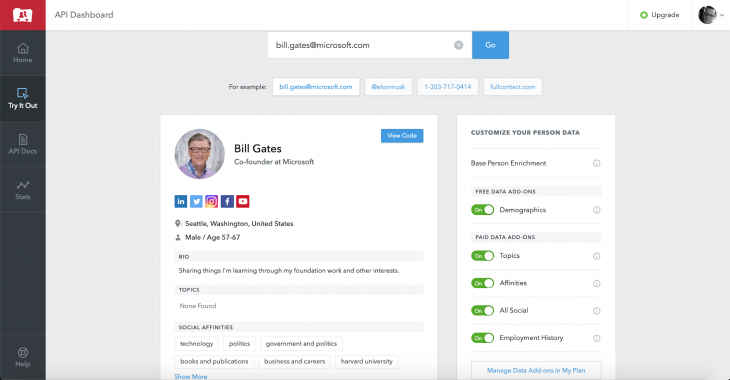The screenshot features a user interface with a light gray background. Starting from the upper left corner, there is a small red rectangle containing a white file folder icon labeled "AI". To its right, "API Dashboard" is displayed in gray text. On the far right, a white "Upgrade" button with a green arrow and a profile icon with a down arrow are visible.

Below this header, a vertical black rectangle runs down the left side, serving as a menu. The menu items, each accompanied by an icon, are as follows: "Home," "Try it out," "API Docs," and "Stats," with "Help" located at the very bottom.

Centered at the top of the gray rectangle is a white search bar, to the right of which is a blue "Go" button. The search bar contains the text "bill.gates@microsoft.com". Directly below the search bar, there's the phrase "For example" followed by three white boxes with blue text inside.

Beneath this section is a white rectangle. At the top left of this rectangle, a profile icon accompanied by the bold black text "Bill Gates" appears, followed by the title "Kodash Founder at Microsoft." In the upper right corner, there's a blue box labeled "View Code." Below, icons for LinkedIn, Twitter, Instagram, Facebook, and a red icon with a white file are displayed in a row, accompanied by small black print.

On the far right side, there is a white vertical rectangle. At the top, it says "Customize your person data," followed by a list of options, each with toggle switches aligned on the left.